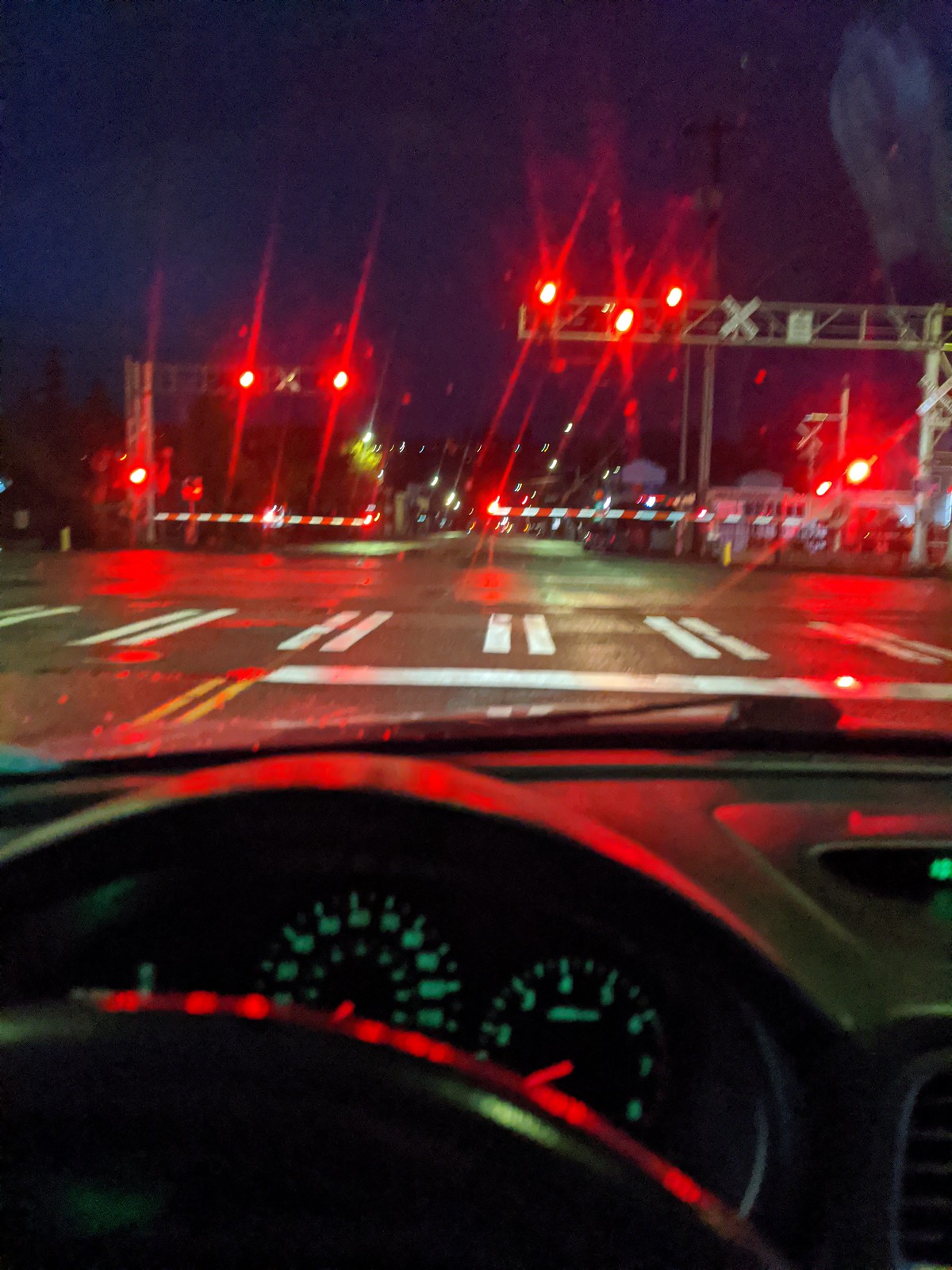The image captures a nighttime scene from the perspective of the driver's seat inside a car. The bottom half of the photo prominently features the car's dark gray-black steering wheel and dashboard. The dashboard elements, including the speedometer and other gauges, are illuminated with light green numbers and red-lit dials, adding a vibrant touch to the interior. Through the windshield, a street and a railroad crossing are visible. The activated crossing is marked by seven bright red lights, with four lights on one side and three on the other, all vividly glowing against the night sky. No train is present, but the scene is set by the visual cues of the activated train stop.